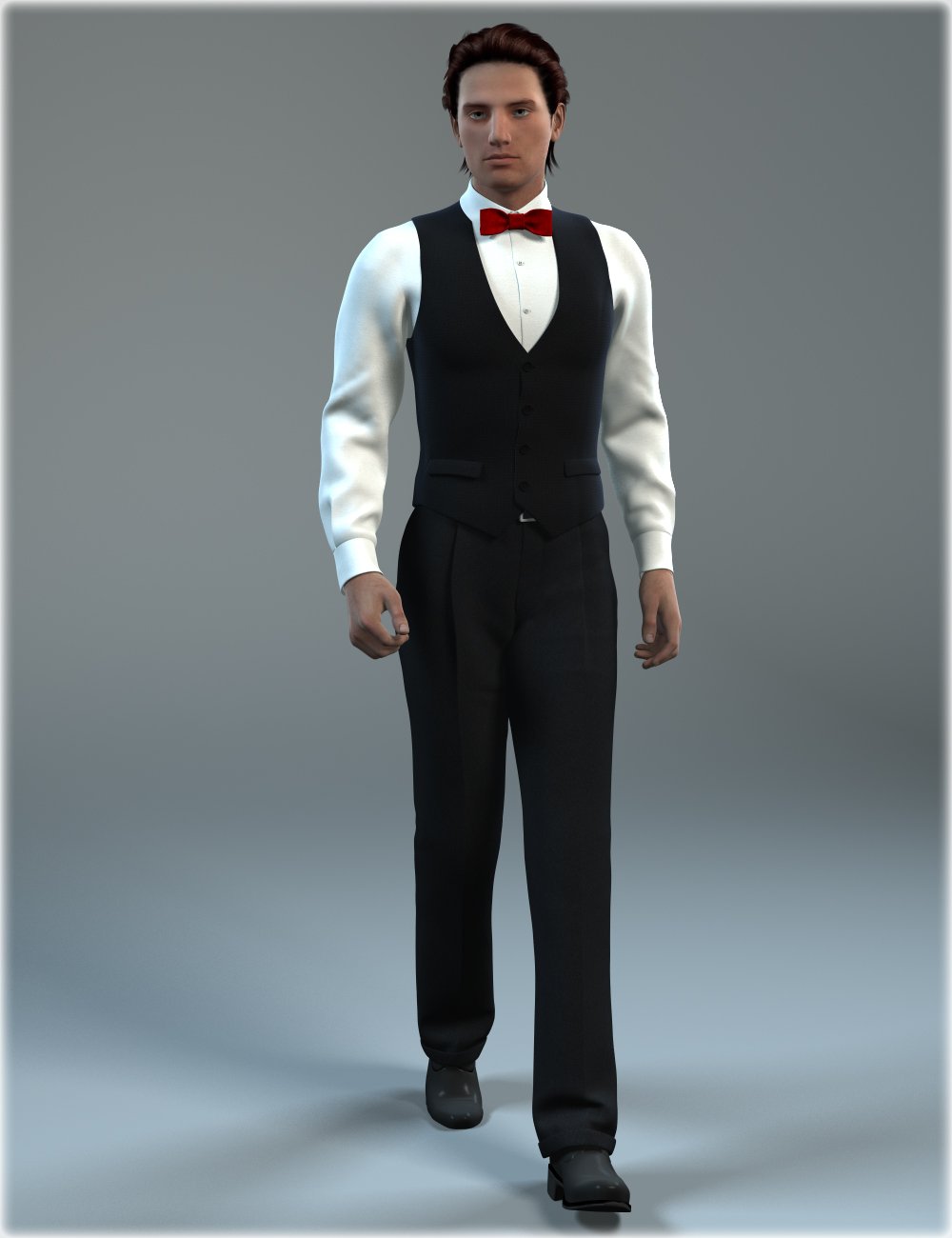The image is a detailed, full-length depiction of a young man who appears to be a character from a video game like The Sims or possibly an AI-generated figure. He has slicked-back black hair and dark skin that would still be considered white. Dressed formally, he wears a white long-sleeved button-down shirt with a red bowtie, a black vest, black dress pants, and black dress shoes. The man is walking towards the viewer with one foot extended forward. His arms are at his sides, and he has a serious expression while looking slightly to the left. The background is a gradient of grayish-green to white, with shadows accentuating the three-dimensional quality of the image, adding to its lifelike yet slightly artificial appearance.